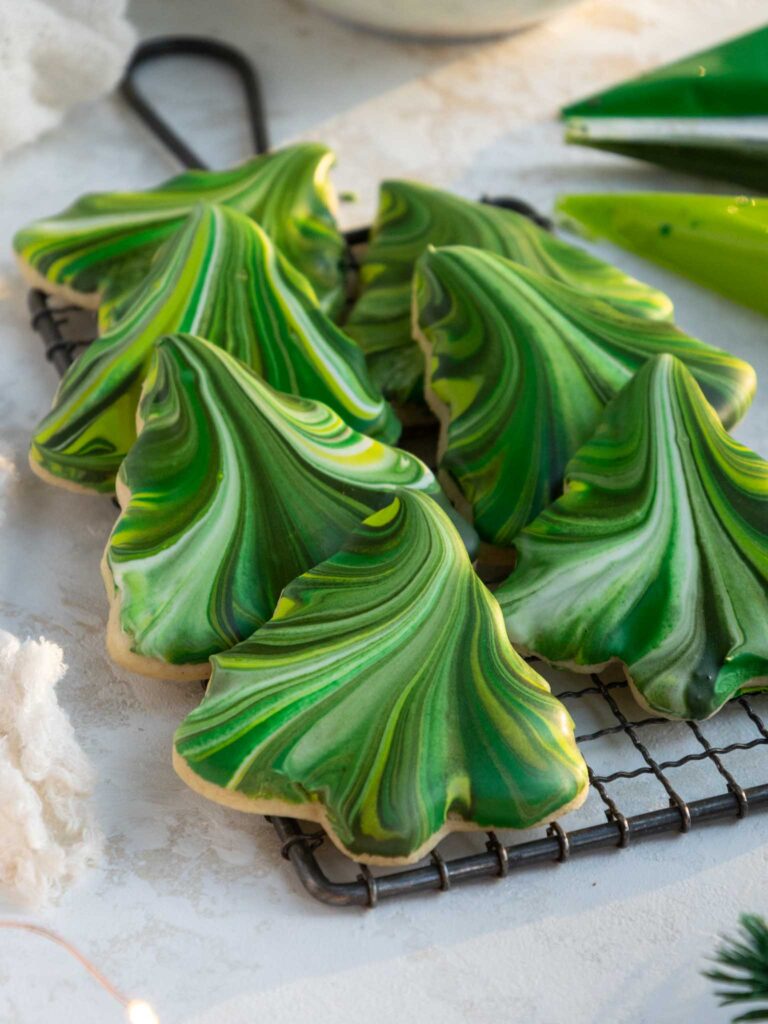In this photograph, a decorative metal grate is placed atop what appears to be a marble countertop with subtle, faded brown designs. Arranged on the grate are seven triangular-shaped cookies, likely shortbread, designed to resemble Christmas trees. These cookies are adorned with marbled green and yellow icing, creating an intricate swirling pattern. To the left of the image, there is a slightly blurry white object, possibly a pastry bag used for decorating. The cookies are carefully positioned with some tilted at various angles, enhancing their tree-like appearance.